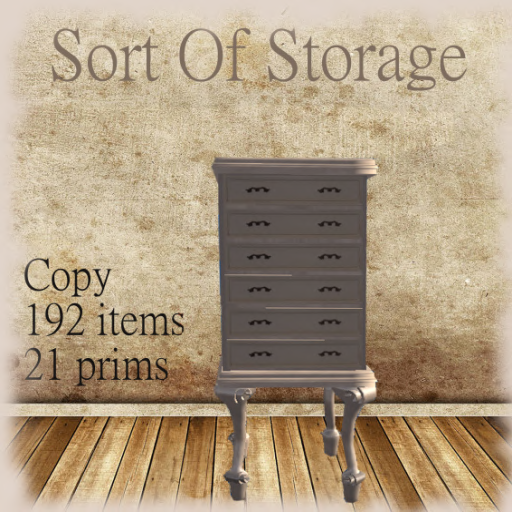This image appears to be an old-fashioned advertisement of a tall, white cabinet or storage chest, featuring six drawers, each equipped with two black handles. The cabinet stands on three prominent legs, which lift it significantly off the ground, although one description mentions casters that suggest mobility, adding to its antiquated charm. The setting includes a worn wooden floor and a weathered white wall marred with brown spots and stains, giving it a rustic, vintage feel. At the top of the image, the phrase "Sort of Storage" is prominently displayed, while to the left side, there are inscriptions indicating "copy 192 items" and "21 prims," lending an odd yet intriguing detail to the scene. The overall tone suggests the image might have been computer-generated, possibly designed to evoke nostalgia or serve as a creative take on a classic furniture advertisement.